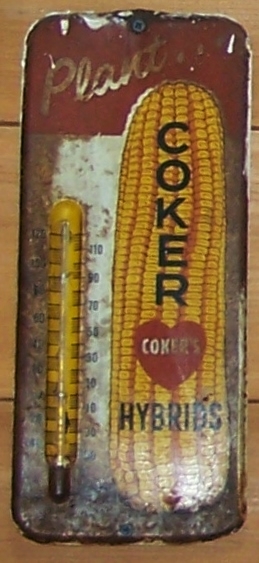The image features a dried corn on the cob, likely field corn, characterized by its densely packed rows of kernels. There are seven distinct rows of vibrant yellow kernels transitioning into a very dried, almost white section towards the bottom. An accompanying yellow object lies next to the corn. Both items rest on a rustic, rectangular tin plate exhibiting a weathered red and white appearance with patches of rust. The tin plate itself is placed on a wooden surface comprised of several planks, suggesting a table or a workbench. Notably, the piece of corn is marked with the text "COKER'S HYBRIDS." The word "COKER'S," spelled out in all capital letters as C-O-K-E-R, is emblazoned within a red heart, while "HYBRIDS" runs horizontally beneath it.